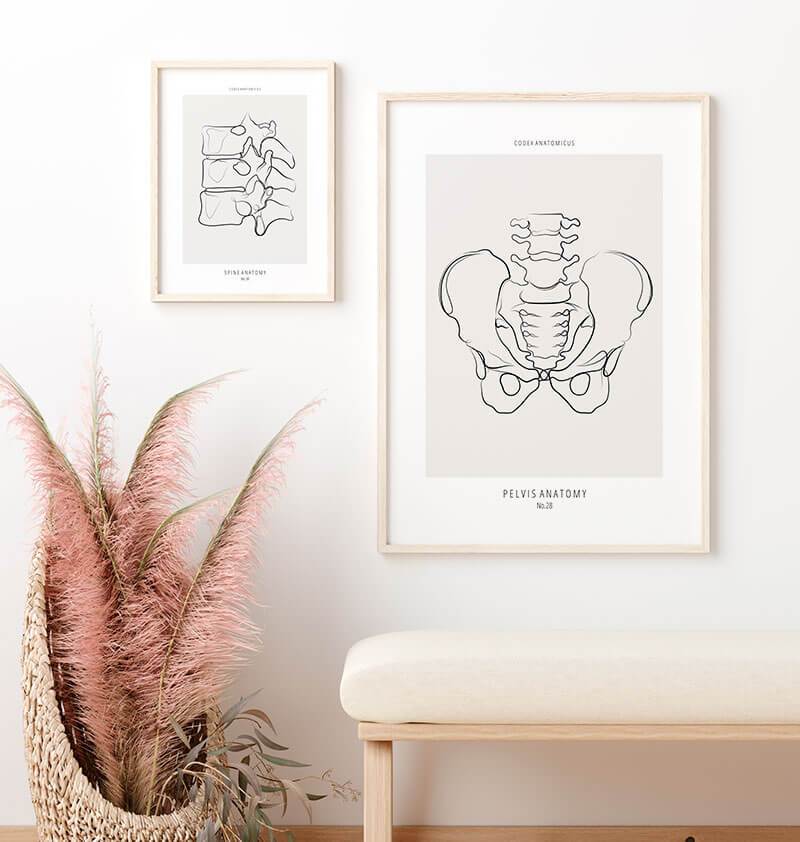The image captures a serene, minimally decorated room with an off-white wall adorned with two art pieces in thin wooden frames. The larger of the two art pieces, labeled "Pelvis Anatomy," features a detailed black and white illustration of the pelvic bone on a beige background with "Code Anatomicus" written at the top and "Anatomy of the Pelvis" at the bottom along with the number "28". To its left is a smaller framed illustration depicting three stacked vertebrae, also in black and white on a beige background. Below the pelvis art, a white bench with a light tan leg is positioned, providing a clean and cohesive look. Adding a touch of organic texture, a woven basket sits to the left of the bench, filled with red, feathery plants.